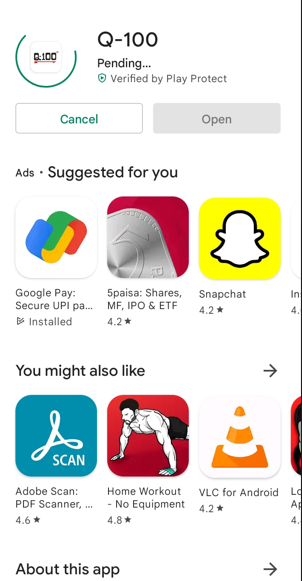This photo captures the installation screen of the Q-100 app from an app store, likely iTunes or Google Play Store. In the upper left corner, there's a white square icon featuring the text "Q-100" in black with a red bar below it, indicating it's the Q-100 app. Surrounding the icon, a green progress arc shows the installation is approximately 80% complete, with the arc forming almost a full circle, missing only the top right section.

To the right of the icon, the name of the app, "Q-100," appears in black font. Below this, the word "Pending..." is displayed, indicating the installation is still in progress. Underneath "Pending," a green shield icon with the label "Verified by Play Protect" signifies that the app has been verified for safety.

Centrally located, there are two prominent buttons: a green "Cancel" button, allowing the user to stop the installation, and a grayed-out "Open" button, which is currently inactive as the app is not fully installed yet.

Below these buttons, an "Ads Suggested for You" section showcases six clickable ad squares. These include:

1. **Google Pay**: A white ad with Google's signature colors—blue, green, yellow, and red.
2. **Five Peja Shares**: An ad with a red background featuring some form of currency.
3. **Snapchat**: A bright yellow ad displaying the iconic ghost logo.

Additionally, suggestions for other apps appear, including "Adobe Scan," "Home Workout," and "VLC for Android," each presented as potential recommendations for the user.